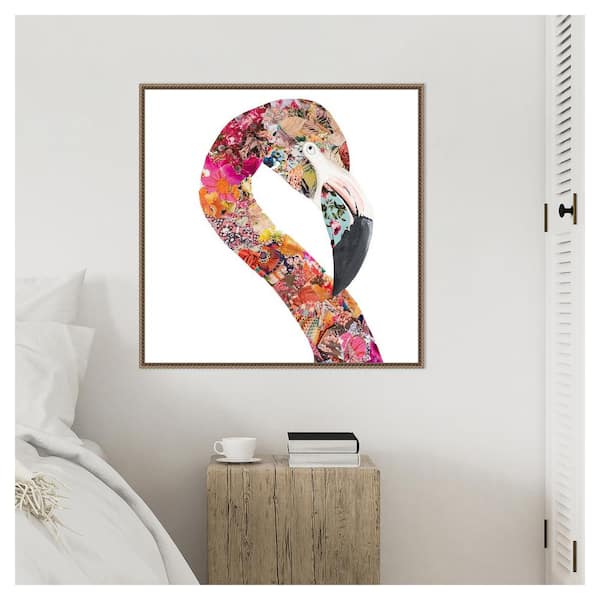This image features a framed poster print displayed on a wall above a wooden nightstand in a cozy bedroom setting. The poster is an artistic depiction of a flamingo, rendered through a collage of various images and graphics. The flamingo's neck and face are intricately composed of multicolored flowers and other objects, blending seamlessly to create a striking visual effect. The bed in the room is adorned with a white blanket and pillow, enhancing the serene ambiance. On the nightstand, there are a couple of books and a coffee cup, contributing to the lived-in feel of the space. Additionally, a closet door with a black knob is visible to one side of the room, adding a touch of detail to this homey scene. This setup mirrors the kind of staged image you might find on retail websites like Amazon, meant to showcase poster prints in a realistic home environment.